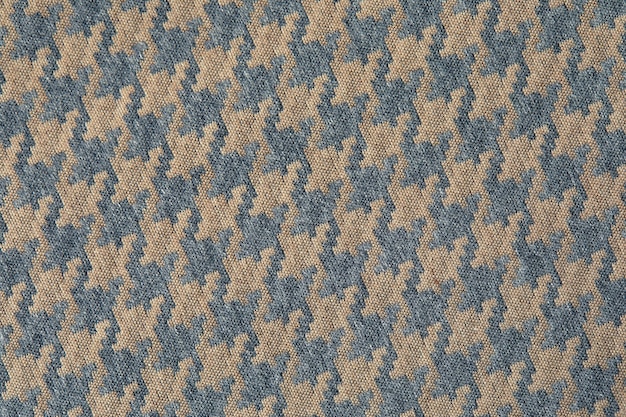The image depicts a close-up view of a finely woven fabric characterized by an intricate, repeating herringbone pattern. The background of the fabric is in various shades of beige, tan, and gold, providing a warm, earthy tone. Interspersed within the pattern are motifs in a bluish-gray hue—potentially representing abstract or dinosaur-like shapes—that run diagonally across the fabric. The design alternates these blue-gray elements with the beige background, enhancing the texture and depth of the fabric. The photograph captures about seven rows across and ten rows down of this tightly knit pattern, which extends to all four corners of the rectangular image. This detailed, cross-hatched arrangement may suggest that the fabric is intended for suiting, given its refined texture and classic herringbone design. The precise use of colors and patterns indicates its potential suitability for high-quality garments rather than more utilitarian items like tablecloths or placemats.